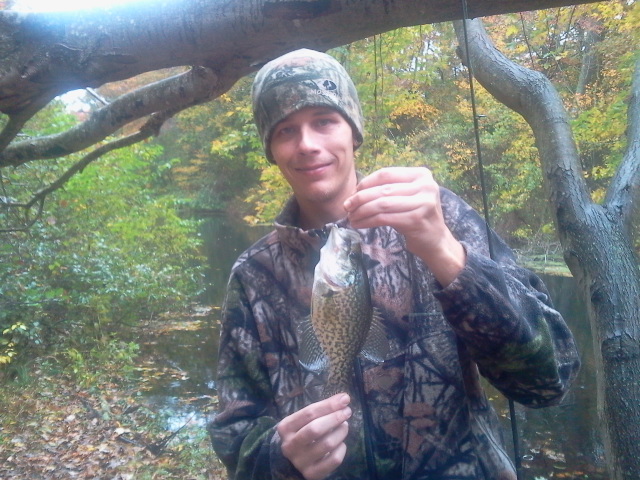The image captures a young man in his early 20s, dressed in a blue, grey, and red camouflage outfit along with a matching beanie pulled down just above his eyebrows. He sports a small, content smile as he proudly displays a small trout, grasping it with both hands—his left hand holding the tail and his right hand grasping the line. The trout is still attached to a black fishing rod tucked between his elbow and his body, situated on the right side of the image. 

Behind him, a serene stream flows, adding a tranquil backdrop to the scene. Over his head, a thick brown and grey branch stretches out, while another tree trunk appears to his right, splitting into one branch that ascends to the left and another that extends to the right. The setting is rich with natural elements, featuring various bushes and trees adorned with green and yellow leaves. The photo, taken in a brightly lit outdoor environment, showcases a range of natural colors from green to brown to grey, encapsulating the essence of a peaceful day spent fishing in the woods. No other people, vehicles, words, or numbers are present in the image, emphasizing the man's solitary connection with nature.